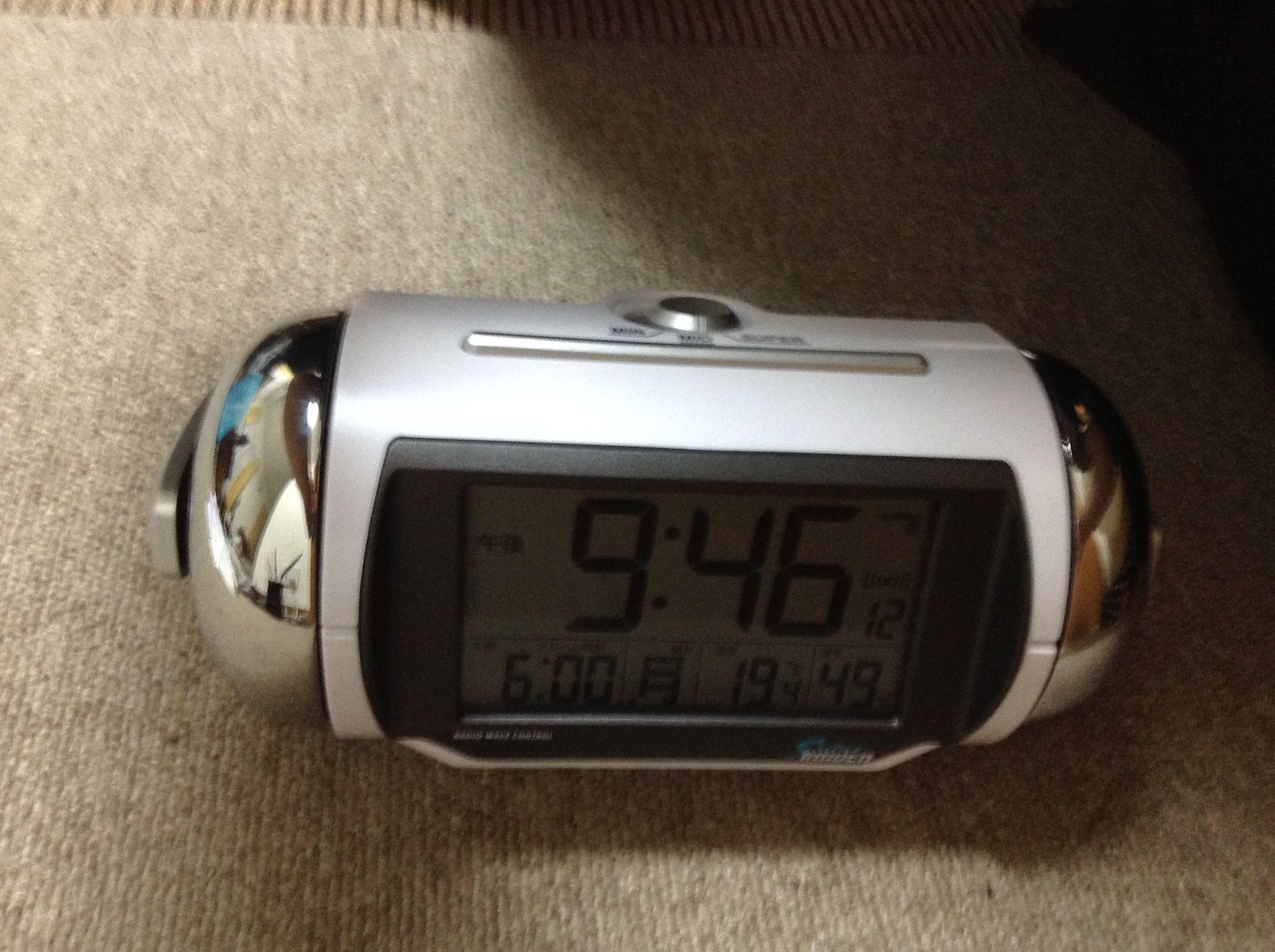This overhead photograph captures a silver cylindrical alarm clock resting on a beige carpet, which features subtle hints of gray and brown. The alarm clock sports a light gray square piece of plastic encircling its center. At the top and in the middle of this plastic strip, there's a prominent raised silver button. Flanking this button, both to the right and to the left, are areas with black writing. Below the writing, a horizontal raised silver bar is positioned. The focal point of the clock is its square black digital display on the front, currently showing the time as 9:46.